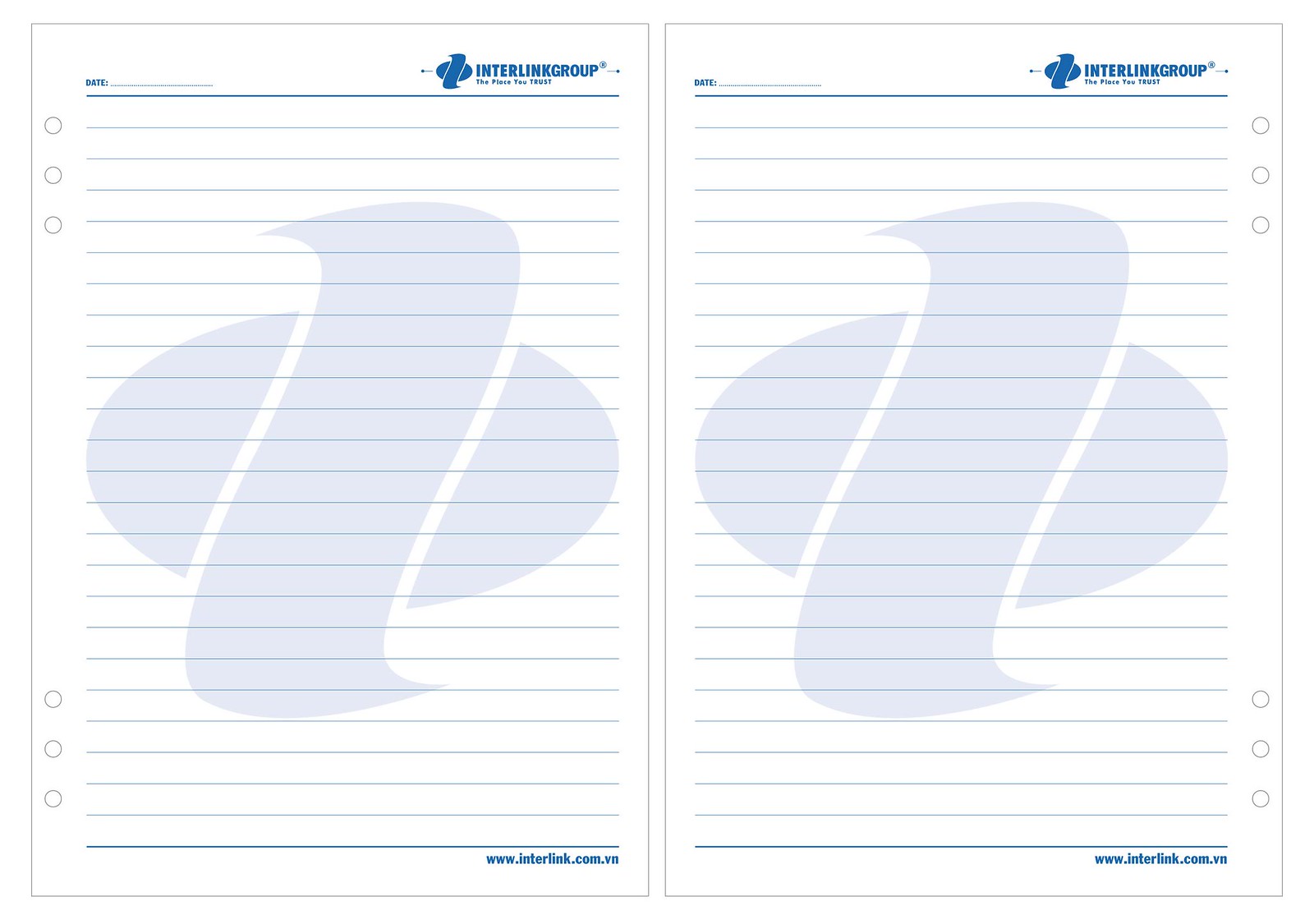The photographic image showcases two nearly identical pieces of white lined note paper, presented side by side. Each sheet features blue lines, creating a structured layout for note-taking or documentation. At the top of both pages, there is a designated space labeled "Date" where the user can fill in the date. Additionally, the Interlink Group's logo, a stylized 'I' resembling an eye within an oval, is prominently displayed in the top right corner, with "Interlink Group" text accompanying it. 

The pages are distinguishable by the placement of three bullet points; they are positioned at the top and bottom left on the left page, while on the right page, the bullet points are mirrored to the right side. A faint watermark of the Interlink Group logo is subtly imprinted in the middle of both sheets, adding a professional touch. Both pages are pre-punched with three holes for easy insertion into binders, with the holes on the left page vertically aligned on the right, and vice versa on the right page.

In the bottom right corner, the contact information is neatly printed, featuring the website address "www.interlink.com.vn." This template, likely intended for business or organizational use, provides a clean and professional format suitable for various documentation purposes.